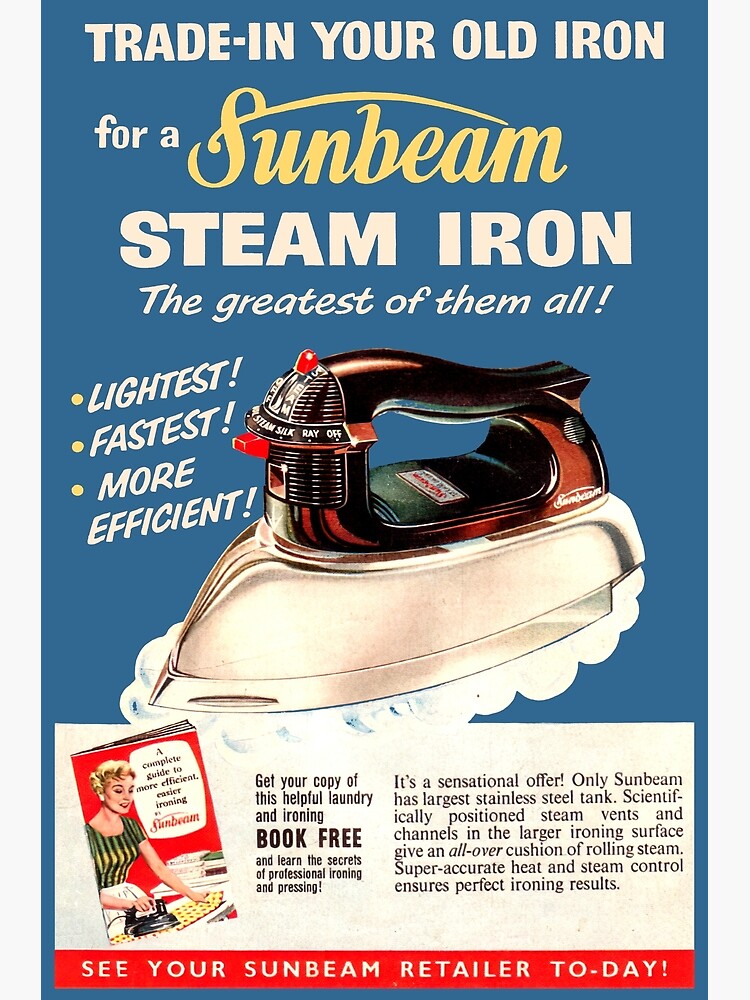This vintage magazine advertisement from the 1950s or 1960s promotes the Sunbeam steam iron, heralded as the "greatest of them all." The top section of the ad features a light blue background with white and yellow cursive letters proclaiming, "Trade in your old iron for a Sunbeam steam iron." It highlights the iron's superior qualities, listing it as the "lightest, fastest, more efficient." The centerpiece of the ad is a detailed drawing of the steam iron, characterized by its red maroon handle and shiny silver bottom emitting steam. Adjacent to the image is promotional text in bold letters emphasizing the product's efficiency. Below the iron illustration, there's an image resembling a magazine cover, featuring a housewife with short blonde hair in a striped shirt ironing, symbolizing the target consumer base. Beside her picture, the text encourages readers to "get your copy of this helpful laundry and ironing book free" to learn professional ironing techniques. The ad culminates with a red banner at the bottom urging, "See your Sunbeam retailer today."